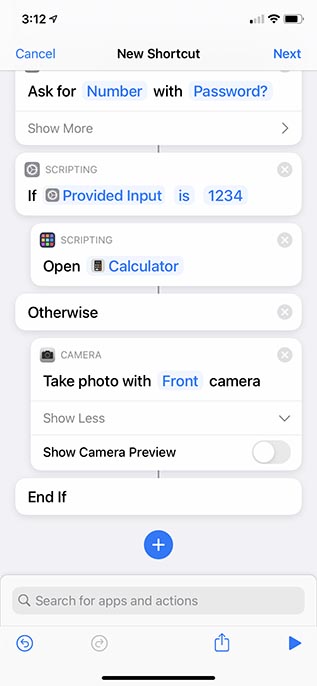This is a detailed screenshot taken from a mobile device displaying a coding application in use. At the top of the screen, common status icons indicate the current time, Wi-Fi connection, network signal strength, and battery life. The bottom of the screen features a navigational menu, including back and forward buttons, a download or upload button, and a play button.

The screenshot specifically captures a window within the application that utilizes a drag-and-drop interface for coding. The script being displayed is partially cropped due to scrolling and is a simple if-else logic sequence. The visible portion of the code reads: 
"Ask for number with password.
If provided input is 1234, 
Open calculator.
Otherwise, take photo with front camera.
End if."

This sequence illustrates a basic conditional statement: if the user inputs the password '1234', the application will open the calculator; if not, it will trigger the front camera to take a photo.